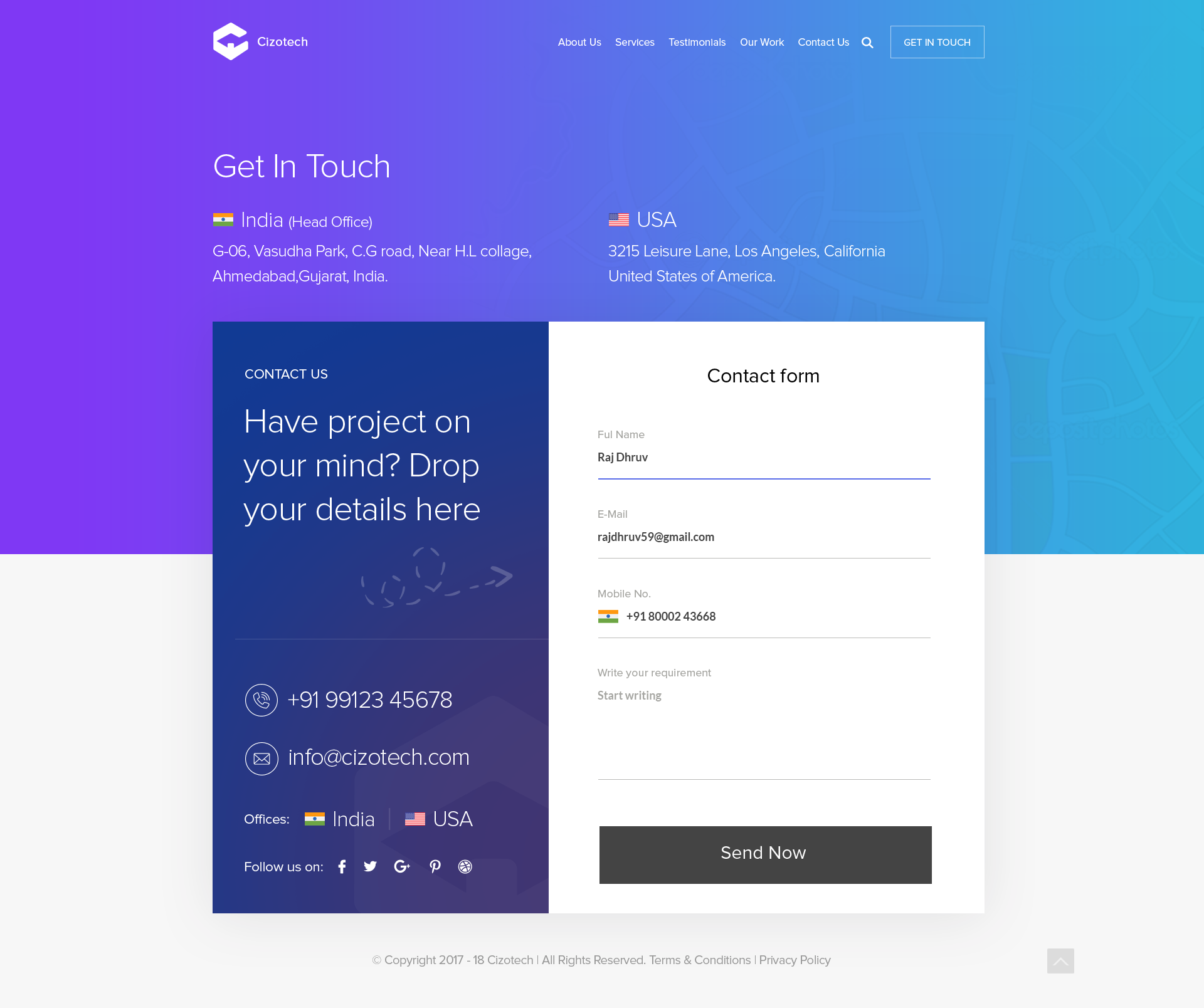The webpage for Sizzotech features a visually striking design incorporating a gradient background that transitions from purple to cyan, going from left to right. At the top, their logo is prominently displayed alongside the company name, "Sizzotech," in bold white font.

The navigation menu, also in white font, includes the following sections: About Us, Services, Testimonials, Our Work, and Contact Us. There's also a search icon, represented by a magnifying glass, and a "Get in Touch" button outlined in a white box to indicate the current page selection.

Dominating the center of the page, the phrase "Get in Touch" is prominently displayed. Below, the contact information for Sizzotech’s offices is provided, denoted by the flags of India and the USA:
- For India (Head Office): G-06 Bazuta Park, CG Road, near HL College, Ahmedabad, Gujarat, India.
- For the USA: 3215 Leisure Lane, Los Angeles, California, United States of America.

A contact form occupies the lower portion of the page, divided into two sections. On the left, a navy blue background hosts a prompt in white text: "Contact Us. Have a project on your mind? Drop your details here." A decorative arrow points towards the form on the right.

Below this text, additional contact details are listed:
- Phone number: +91 991245678
- Email: info@cizotech.com

Social media icons for Facebook, Twitter, Google Plus, and Pinterest are also displayed, along with another icon that is indistinguishable.

On the right side, the contact form appears within a white box. It is partially filled out with the following information:
- Full Name: Raj Dhruv
- Email: rajdhruv59@gmail.com
- Phone Number: +91 812345678

An area designated for writing a requirement remains blank, labeled "Start writing here." The form concludes with a black button featuring the text "Send Now" in white.